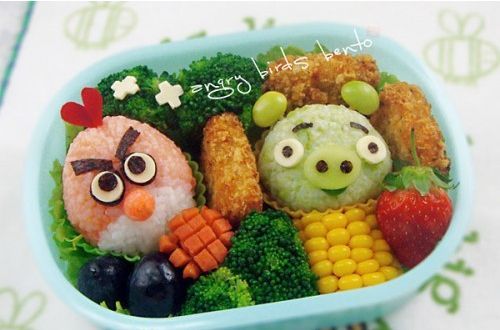This image showcases a meticulously crafted and adorable bento box lunch for a child, themed after the popular game Angry Birds. The blue bento box sits atop a white placemat adorned with bumblebees. Inside the container, the phrase "Angry Birds Bento" is visible, setting the stage for the creative culinary art within. The bento box features various rice formations, vividly colored to resemble the iconic Angry Birds characters. One character, a red Angry Bird, has been fashioned with red rice for the body, with white rice below and detailed with seaweed eyebrows and accents that creatively use a bit of carrot for the beak and Oreo-like pieces for the eyes. Another character, a green pig, has a face made of green rice, with green grape ears, a grape nose accented with raisins for nostrils, and additional details formed from various fruits and vegetables.

The box is a vibrant medley of nutritious ingredients, including broccoli, juicy strawberries, large black grapes, corn, cut-up carrots, and possibly some chicken nuggets or potato cakes. The attention to detail is evident in how the vegetables, such as lettuce and potatoes, are ingeniously used to mimic the characters' features, bringing them to life. This inventive bento box is not only visually appealing but also packed with a variety of healthy foods, sure to delight any child at lunchtime.